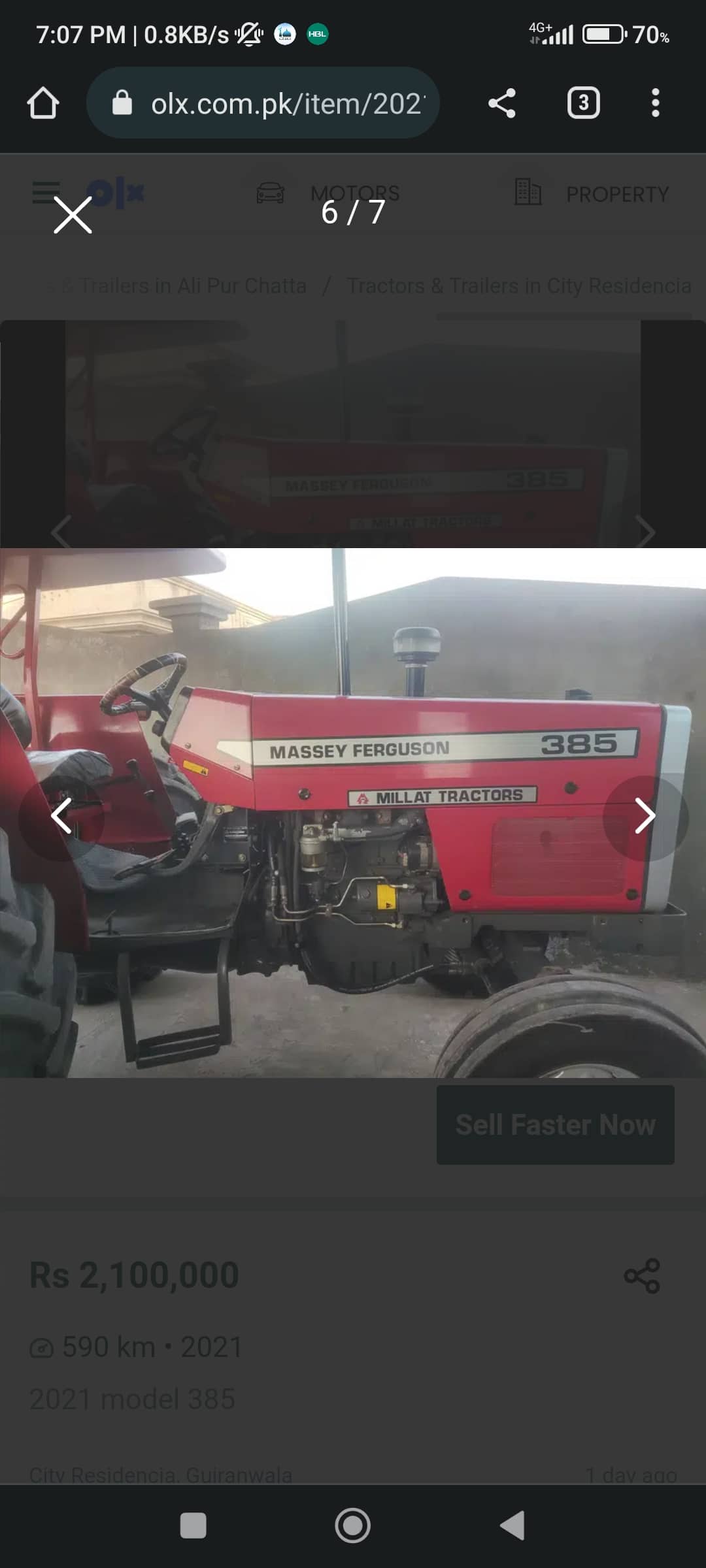This screenshot captures a web-page displaying a photo gallery interface. Positioned at the top-left corner is an X button for closing the gallery. Centrally aligned at the top, the text "6/7" indicates that the current image is the sixth out of a total of seven in the gallery. Just below this header, two arrow buttons are visible on either side of the image, allowing navigation through the gallery.

The current image showcases a red tractor with a pronounced square body design. A white banner emblazoned with "Massey Ferguson 385" runs along its side. 

Above the URL bar, the website address reads "olx.com.pk/item/202." In the browser interface, a Home button is visible to the left, followed by the Share, Tabs, and More Info buttons on the right.